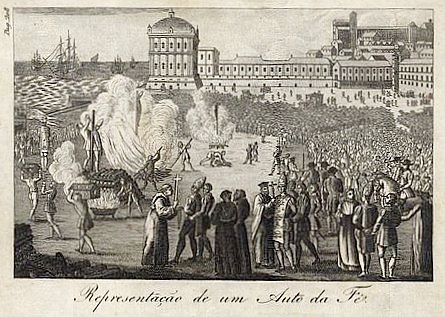This image, a black-and-white photograph of an old, hand-drawn illustration on an off-white canvas, portrays a grim medieval scene. In the foreground, several figures, drawn in a cartoonish style, are depicted. Prominently, there are religious figures wearing large, pointed hats and holding crosses, including a priest with a large cross. These religious figures stand near individuals who appear to be condemned, possibly hinted at by smoke rising around them, suggesting they are being burned at the stake. To the right, men on horseback can be seen, adding to the chaotic atmosphere.

In the center of the foreground, several people are visibly gathered, possibly in the throes of some sort of religious persecution or execution, observed by an extensive crowd that extends into the background. Hundreds, possibly thousands, of spectators fill the scene, creating a sea of people that seems to be witnessing this gruesome event. Some members of the crowd appear to be carrying items to the fires, while others perhaps march towards the site of the burning.

The background is dominated by the silhouette of large structures, potentially castles or town buildings, hinting at a grand medieval setting. On the left side of the image, the masts of tall ships are visible, indicating a nearby body of water, possibly the sea. Intriguing cursive text at the bottom of the image reads "representation de om auto de frae," suggesting the drawing might depict an Autos de Fé, a historical public act of penance during the Spanish Inquisition.